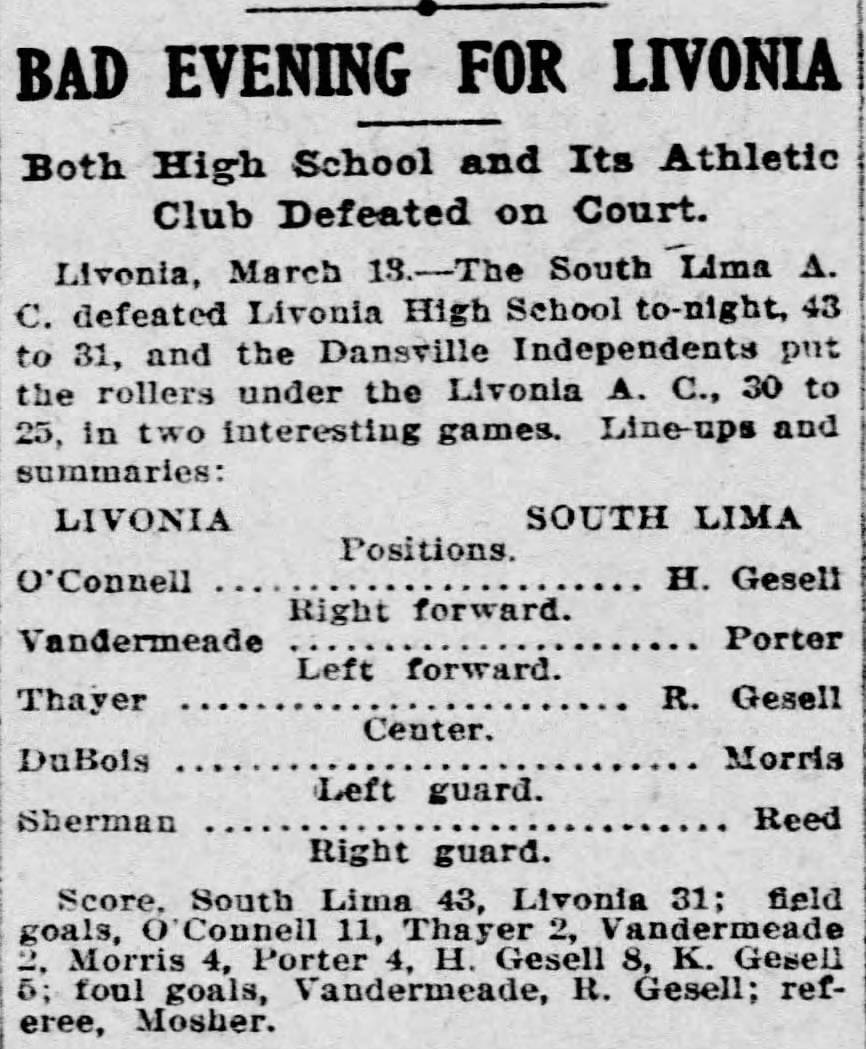This image shows an old newspaper clipping with the headline "Bad Evening for Livonia," summarized under the sub-headline "Both High School and Its Athletic Club Defeated on Court." Dated March 13th from Livonia, the article details that South Lima A.C. triumphed over Livonia High School with a score of 43 to 31, while the Dansville Independents overcame Livonia A.C. 30 to 25 in two engaging basketball games. The clipping includes lineups and summaries, listing Livonia's starting players on the left and South Lima's on the right, positioned according to their roles—right forward, left forward, center, left guard, and right guard. Below this, the scores and statistics of the game are provided, including notable performances such as O'Connell's 11 field goals and H Geisel's 8 field goals, with fouls noted for players like Vandermeer and R Geisel. The overall presentation and typeface suggest the clipping is from an older publication, lending a sense of historical context to these local sports outcomes.